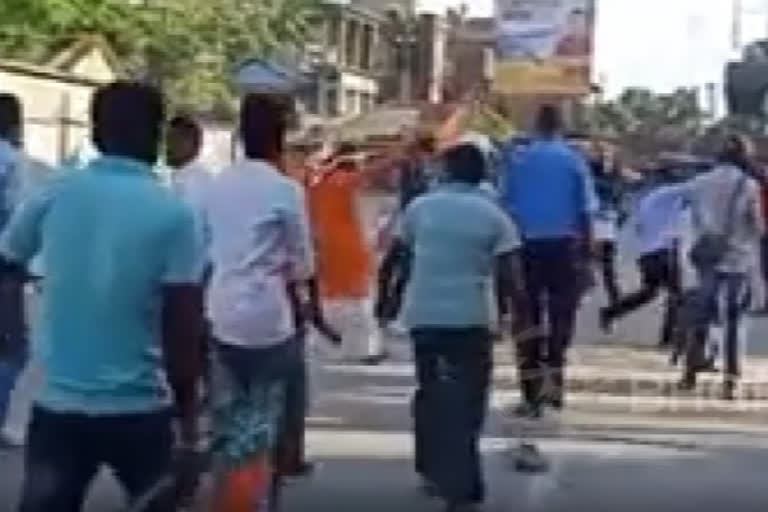This blurred photograph captures a bustling city street scene with numerous people prominently visible in the foreground. Due to the lack of clarity, specific features are hard to discern, and visual details are somewhat ambiguous. The backdrop features an indistinct structure that could either be a building or possibly a mountain.

To the far left, a tan-colored house is partially visible, accompanied by some trees behind it. A man on the far left, with his back turned, is walking away wearing a light-colored, short-sleeved shirt and jeans. He appears to be holding something in his right hand, though it is indistinguishable due to the blurriness.

Ahead of him, another individual, clad in a white long-sleeved shirt and jeans or trousers, is also walking away. In the center of the image, a person in a medium bluish-green short-sleeved shirt is visible, exhibiting darker arms and dark-colored trousers, also moving away from the camera.

To his right, another figure wears a medium blue short-sleeved shirt with darker pants, similarly captured from behind as they walk away. On the far right, the next most visible person, potentially a woman, sports a lighter top and dark jeans or pants. She carries a crossbody purse with the strap over her right shoulder, hanging on her left side. All depicted individuals have their backs facing the camera, creating a unified sense of movement away from the viewer.